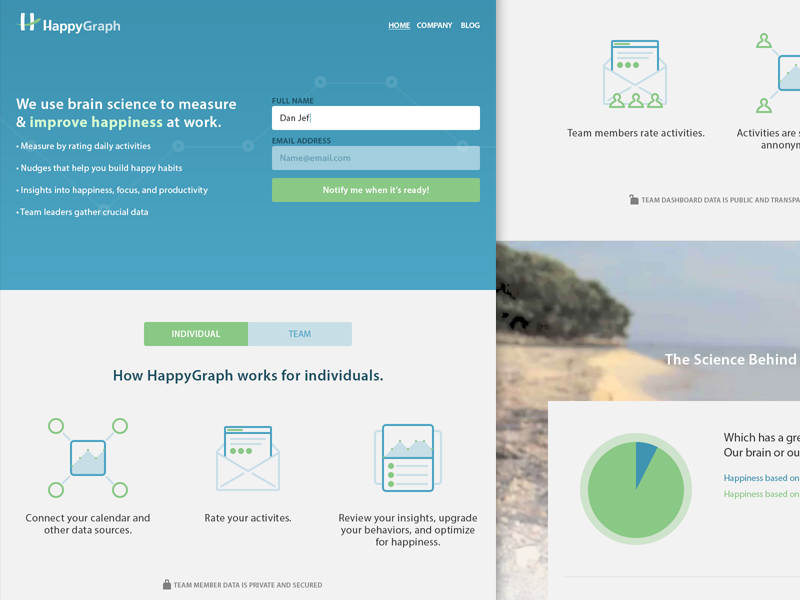**Caption:**  
This screenshot captures the homepage of a website called "Happy Graph." The website's name is prominently displayed in white text on a blue background in the upper left-hand corner, accompanied by their logo featuring a white "H" with a green curved line forming the center. On the upper right-hand corner, there are white navigation links labeled "Home," "Company," and "Blog."

The left-hand side features a tagline in white and green text that reads: "We use brain science to measure and improve happiness at work." Below this, four bullet points detail the services offered:
1. Measured by rating daily activities.
2. Nudges that help you build happy habits.
3. Insights into happiness, focus, and productivity.
4. Team leaders gather crucial data.

On the right-hand side, there is a form for users to fill out. The form prompts for the "Full Name," shown in a white rectangular bar containing the example "Dan Jeff." Below it is a field for "Email Address," depicted in gray with the placeholder "name@email.com." The final field is a green rectangular button displaying "Notify me when it's ready" in white.

Beneath this form, two buttons on a white background allow users to select between "Individual" in green and "Team" in gray. A bold black heading states, "How Happy Graph works for individuals." 

At the bottom, three large grayish-green icons illustrate the process:
1. A square with dots in each corner, labeled "Connect your calendar and other data sources."
2. An envelope with a piece of paper, titled "Rate your activities."
3. A paper with a data graph, accompanied by three lines of text with green dots, stating, "Review your insights, upgrade your behaviors, and optimize for happiness."

To the right, an ocean image with white text partially off-page reads, "The science behind." Below, on an off-white background, a green dot with a dark blue pie wedge says, "which has a." Above this, another envelope icon notes, "Team members rate activities," and mentions anonymous activities along with small green Parcheesi-like people icons.